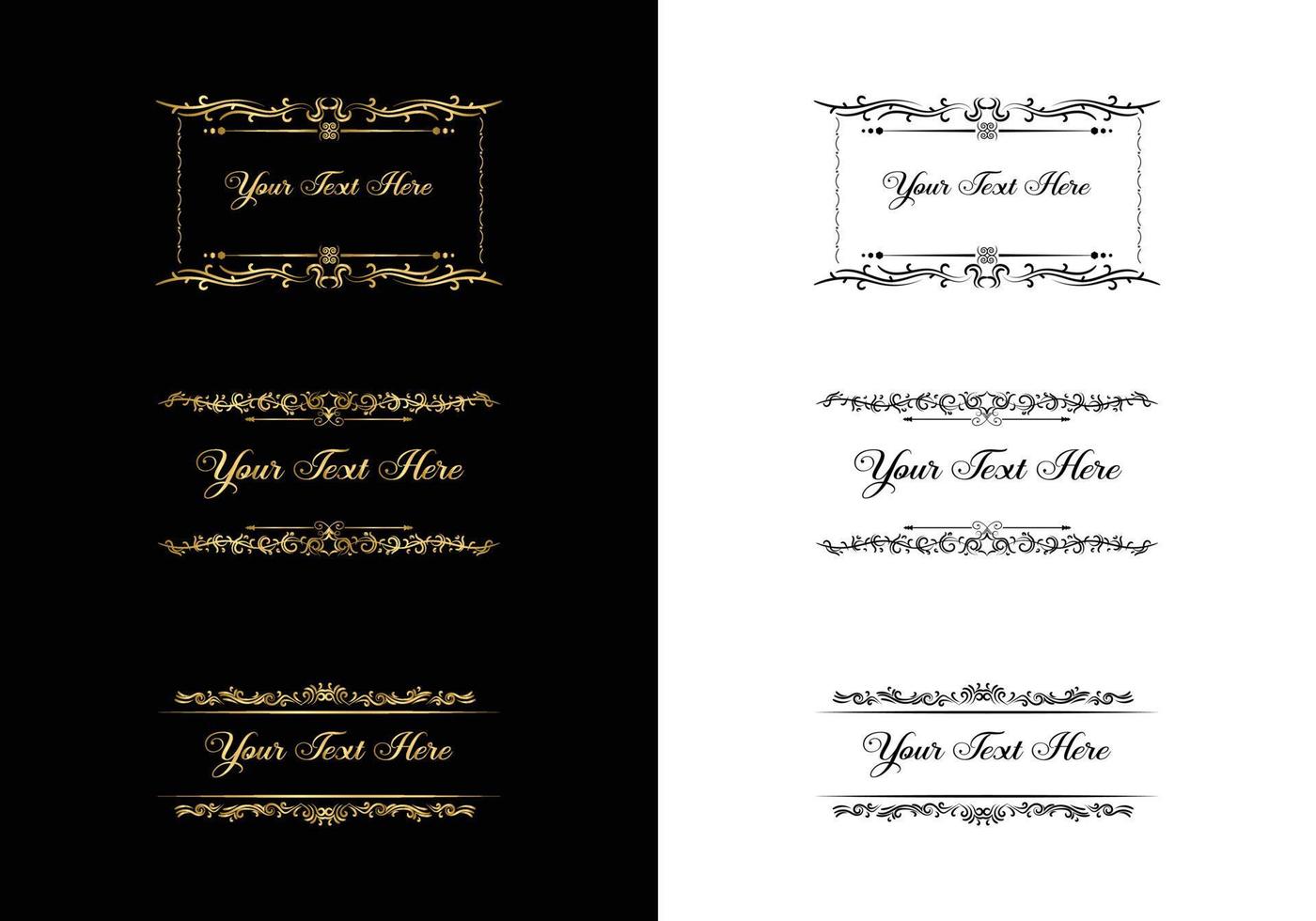In the image, we see a vertically rectangular print piece that is divided into two halves, mirroring each other. The left half features a black background adorned with gold text, while the right half has a white background with black text. Both sections display identical layouts, with ornate decorative elements framing the top, middle, and bottom, creating a sophisticated and elegant look. Each section prominently displays the placeholder text "Your Text Here" in cursive. The topmost section has ornate decorations above and below the text, the middle section follows similarly with its own decorative accents, and the bottom section mirrors this design. The overall design suggests a customizable template, likely intended for personalized messages or invitations. The black and gold combination on the left side offers a luxurious and striking appearance, whereas the black and white combination on the right provides a more classic and simple look.